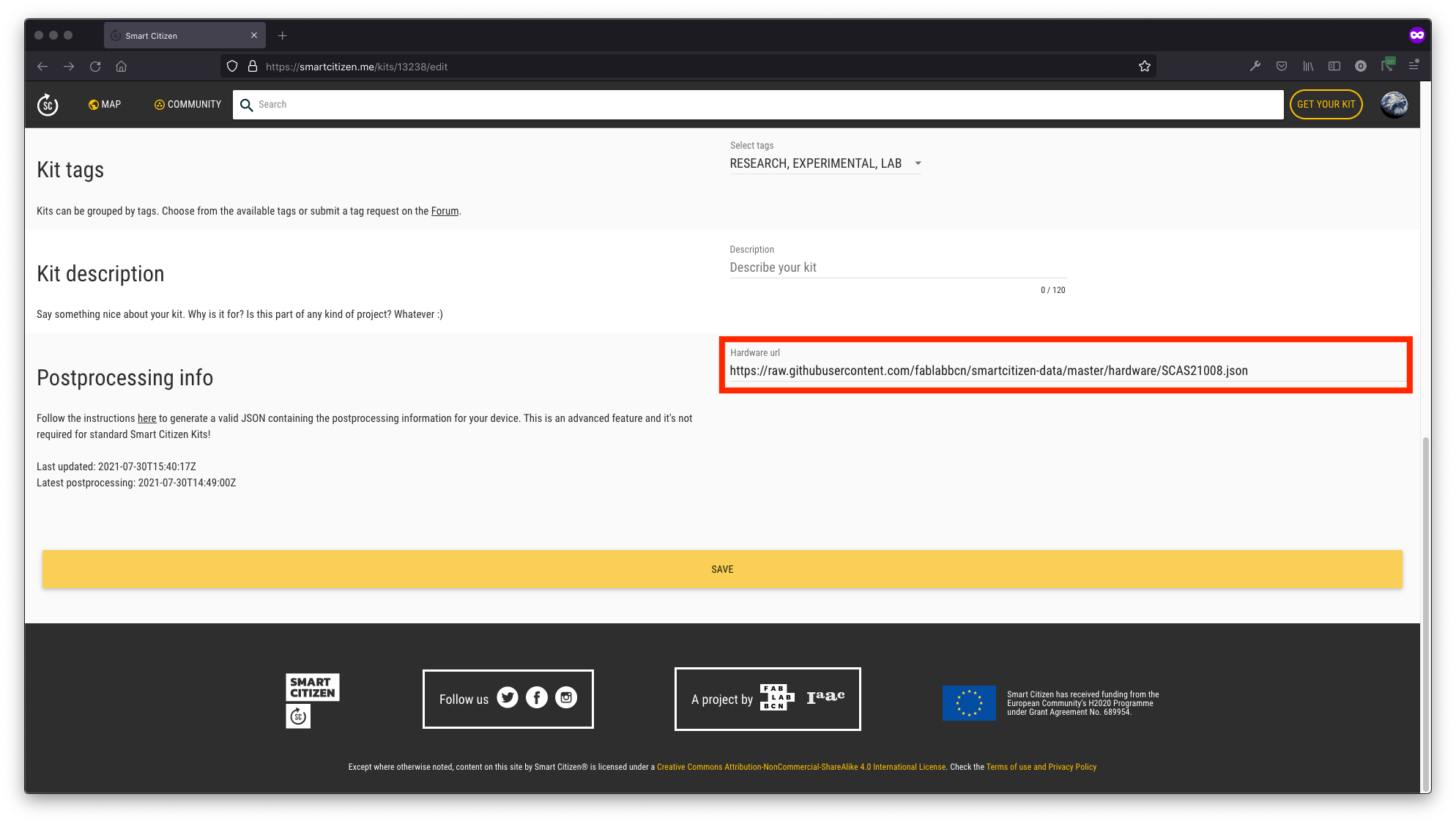A screenshot displaying a webpage from HTTPSmartCitizen.me. At the top of the page, the navigational elements include options for a map, community, and a search function. Midway down, notable headings such as "Kit Tags," "Kit Description," and "Post Processing Info" are present. The "Select Tags" section on the right-hand side prompts users to choose from available tags or submit a tag request through a form. The "Kit Description" section invites users to describe their kit in up to 120 characters, though no description has been entered yet. The "Kit Tags" section explains that kits can be grouped by tags, providing instructions for selecting or requesting new tags. Towards the bottom, the page features social media follow links for Twitter, Facebook, and Instagram. The footer of the page credits FabLabBCN as the project creator, emphasizing its novelty and the user's unfamiliarity with such kits.